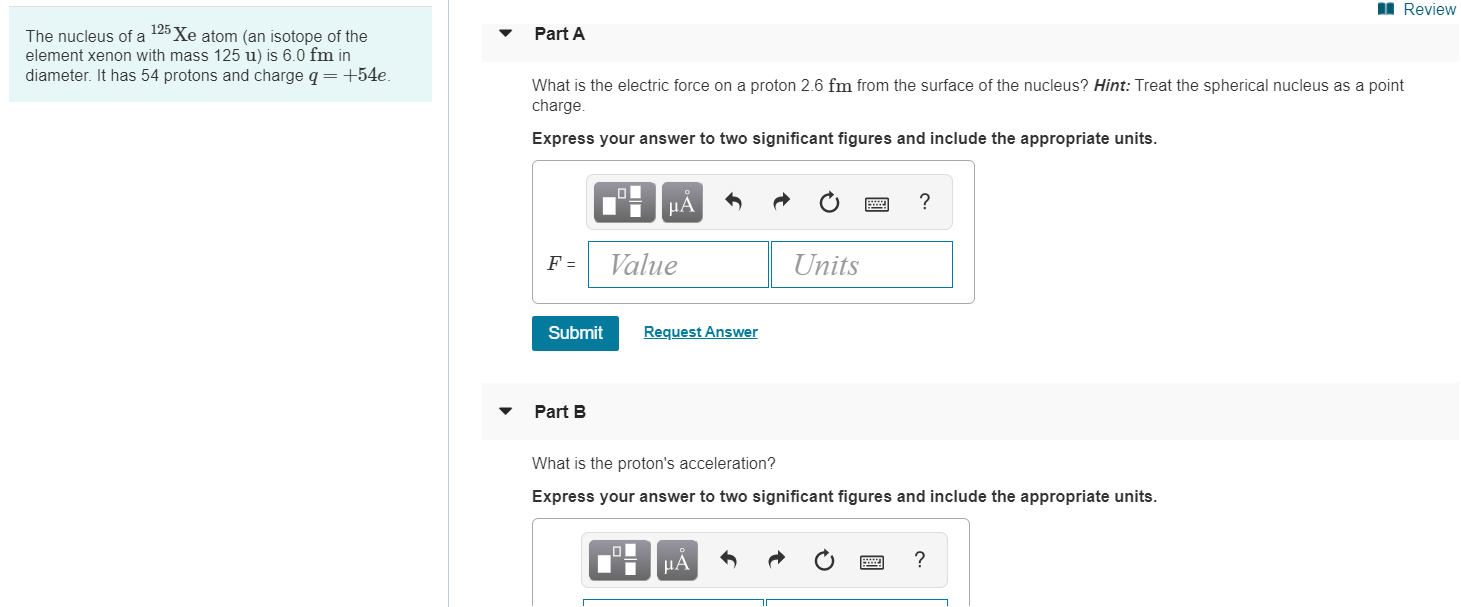The image depicts a straightforward screenshot of a website designed in a minimalist style with a limited color palette featuring cream, blue, gray, black, and white tones. On the left-hand side, towards the top, there is a blue text box containing black text. The text provides information about the nucleus of a 125 Xe atom, specifying that it is an isotope of xenon with a mass number of 125 and a diameter of 6.0 femtometers (fm). The nucleus is described as having 54 protons and a charge of Q = +54e.

To the right, the page is divided into two parts, A and B. Part A presents a question that asks for the electric force acting on a proton positioned 2.6 femtometers from the surface of the nucleus. The problem suggests treating the spherical nucleus as a point charge and requests the answer to be expressed to two significant figures, including the appropriate units. Below this question, there is an arrow pointing downwards to a text box where users can enter their answers. This section also includes a submit button labeled "Submit Form" and an option to request the correct answer.

A section labeled "Review" is situated at the top of the page, which users can click for further assistance. Below Part A, there is Part B, which poses another question: it asks for the acceleration of the proton (presumably as it moves 2.6 femtometers from the nucleus). Similar to Part A, it asks for the answer to be provided to two significant figures and with appropriate units. Part B also includes a text box for input, although the screenshot cuts off the lower part of the text box slightly.

Overall, the website appears to serve an educational purpose, functioning as both a study guide and an interactive testing platform.